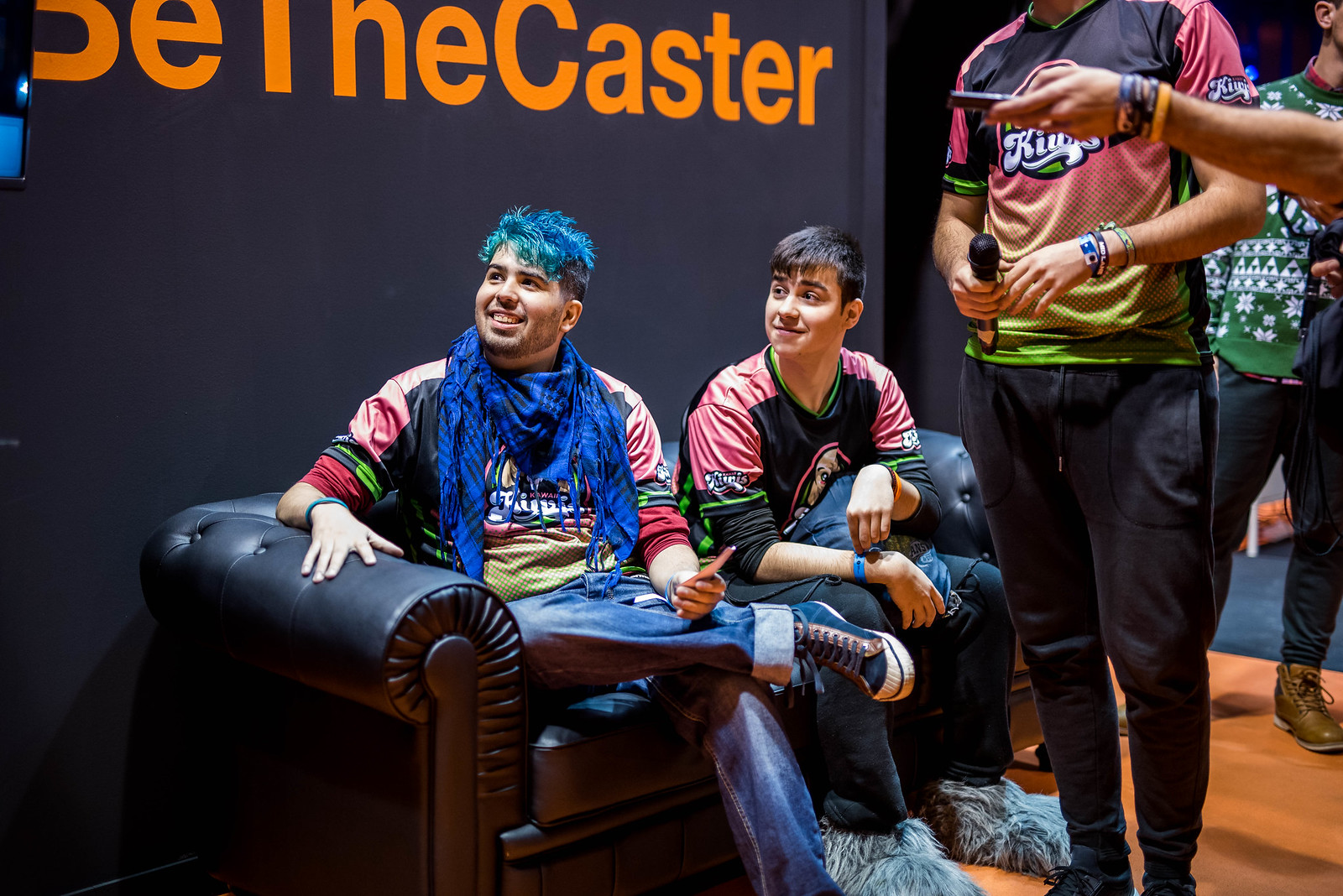The photograph depicts a lively scene at a convention or event, characterized by vibrant colors and an energetic atmosphere. Central to the image are two young men seated on a loveseat-like bench, both wearing striking jerseys in shades of pink, lime green, and orange embellished with a white logo that reads "Kings." The man on the left sports bright blue hair, complemented by a blue scarf and blue jeans. His companion, with short brown hair, is also clad in a "Kings" jersey, blue jeans, and whimsical, hairy footie slippers. Both appear to be looking to their right, smiling.

Behind them, the black wall features large, bright orange letters stating "be the caster," indicating some motivational or directive theme possibly related to the event. Standing to the right of the seated men is another individual holding a microphone, seemingly addressing the crowd. Additional figures linger in the background, some partially obscured but clearly engrossed in the unfolding activity. The setting suggests a spacious interior with wooden floors and sections of carpet, adding to the ambiance of a bustling public gathering.